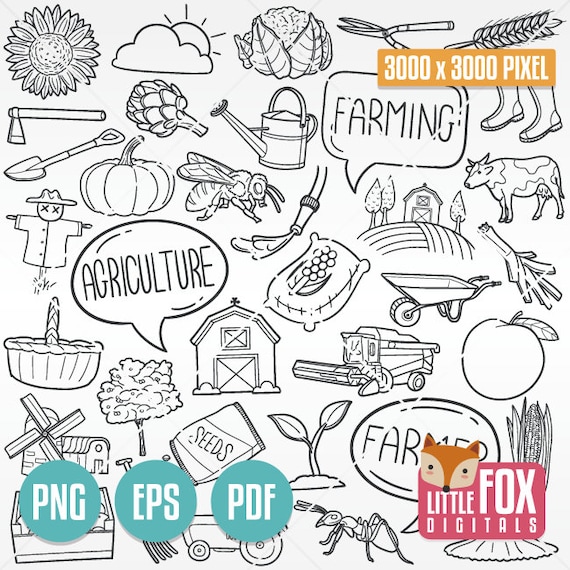This image is a highly detailed, black-and-white illustration reminiscent of a coloring book page, rich with farming and agriculture-themed icons. The central section features a variety of icons including a scarecrow, bee, watering can, barn, seeds bag, wheelbarrow, cow, apple, pumpkin, farm boots, secateurs, windmill, farm machinery, and vegetation like corn and an apple tree. Two speech bubbles label “farming” and “agriculture” respectively. Additional details include a sun peeking through clouds, a rustic scene with a farmhouse and trees, and a sprout emerging from the ground. The upper right corner specifies the image resolution as 3,000 by 3,000 pixels in white text on an orange background. The bottom right corner features the logo "Little Fox Digitals" in white text on a red background, accompanied by a colorful cartoon fox with an orange and pale brown face. On the bottom left, three green circles labeled PNG, EPS, and PDF indicate the available downloadable formats.